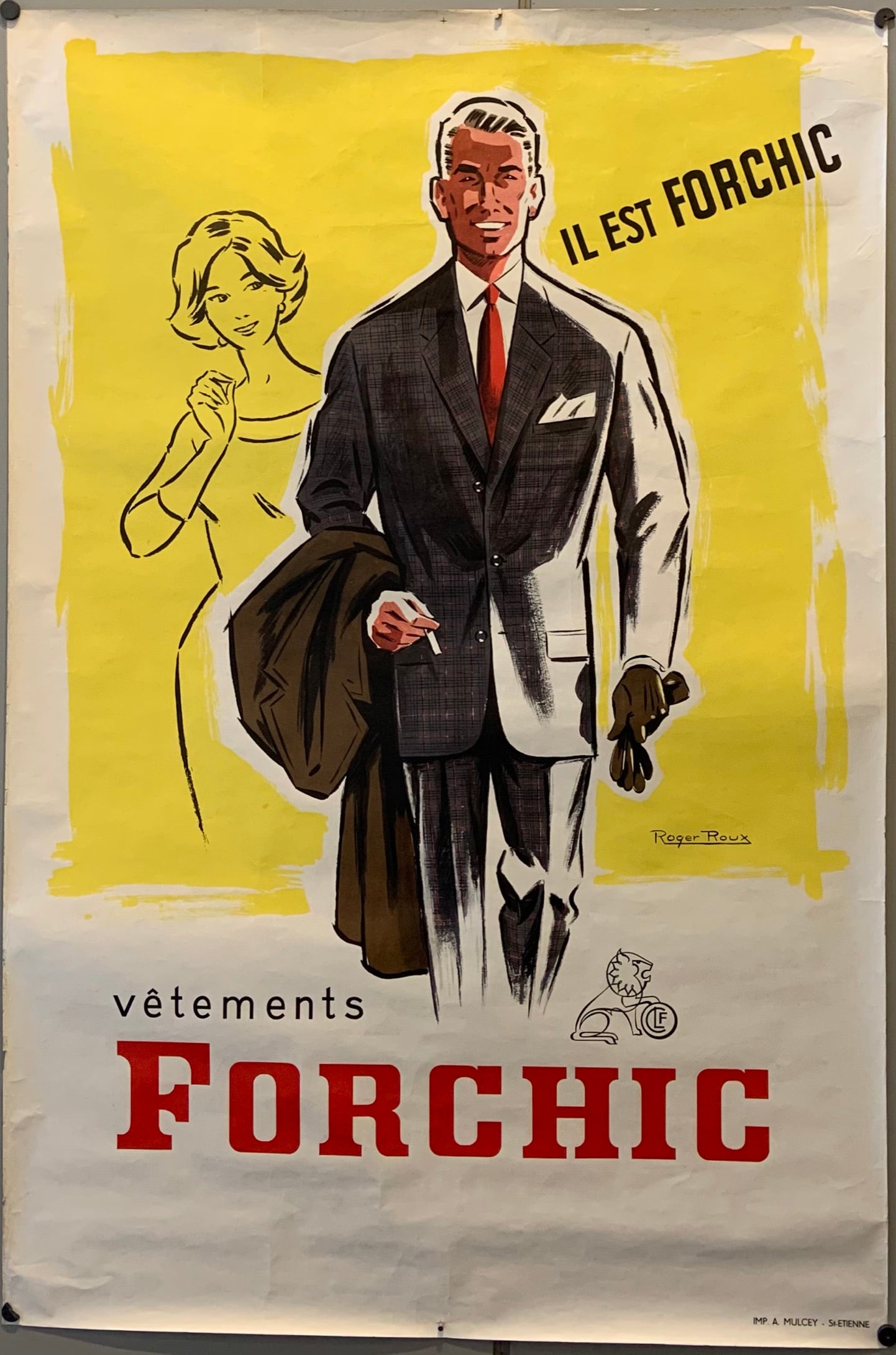The image depicts a vintage poster with a distinct mid-20th-century style, possibly from the late 1940s to the 1950s. The background is beige, and there is a broad yellow block of paint creating a vibrant backdrop. At the center, a rich-looking man is prominently featured. He is dressed in a black suit with a white shirt and a red tie, exuding a confident demeanor with a big smile on his face. His hair, streaked with black and white, complements his sophisticated look. Draped over his left arm is an overcoat, and he appears to be carrying a pair of gloves in his right hand. There's this silhouette of a young girl to his left, drawn in a pencil-like sketch, who looks at him admiringly with a hand near her lips, expressing a sense of marvel.

The poster displays French text: diagonally across the yellow block is the phrase "Il Est Fourchique" in black font, which suggests chic or elegant fashion. Below this, against the wrinkled beige background, it says "Vetements" in black font, translating to "Clothes." Below this text, a lion with a crest symbolizes the Fourchique brand, followed by the brand name "Fourchique" in prominent red lettering. The lower right corner of the poster contains some additional text, but it is not legible. The overall look of the poster is sophisticated and stylish, mirroring the confident appearance of the man featured.